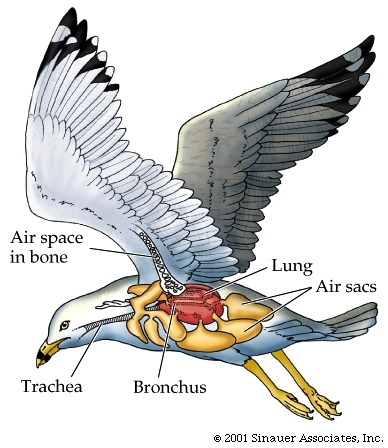This image is an anatomical illustration of a seagull depicted in flight. The bird, white with black-tipped feathers and plume, has its yellow legs and claws extended downwards. The seagull features a distinctive yellow beak with a black stripe. The illustration, done in a cartoon-like yet realistic style suitable for a textbook, provides a detailed cross-section of the bird's internal anatomy, highlighting various organs and structures. Labels point to the trachea, noted as the bronchus in the center, the lungs which are colored red, the air sacs which have a yellow-brown hue, and the air spaces within the bones, especially evident in the wings. The feathers are illustrated to show their orientation in flight, enhancing the realism of the scene. At the bottom, a copyright notice reads "Copyright 2001, Seinauer Associates Incorporated."